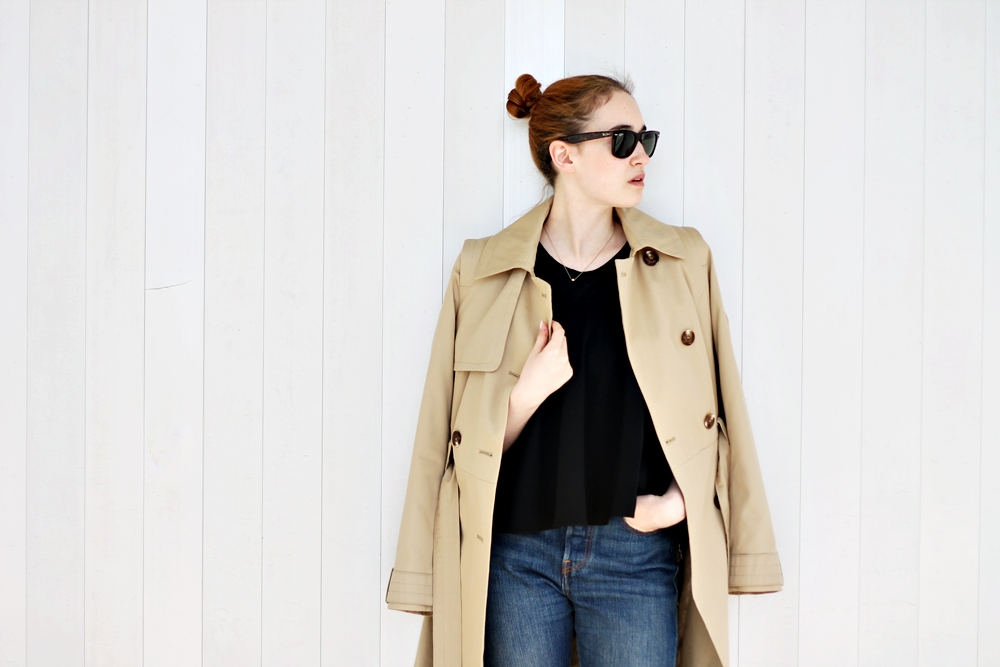A young woman with fair, white skin and red hair pulled back into a bun stands confidently in front of a white plank wall, composed of both pristine and slightly faded wooden panels. She is wearing large, black sunglasses that resemble Wayfarers, and her lips, painted pink, are slightly parted to reveal the top of her teeth. Around her neck is a delicate gold necklace that rests on a black t-shirt. Over her shoulders drapes a light brown trench coat, adorned with several dark brown buttons—three on the left side and at least one visible on the right—that remains open to show her full outfit. Her left hand is casually tucked into the pocket of her dark blue jeans, while her right hand grips the collar of her trench coat. She gazes off to her right, adding a contemplative air to her poised stance. The overall bright and light-toned setting suggests that the photograph was taken during the day, possibly for a fashion advertisement, showcasing her ensemble in vivid detail.